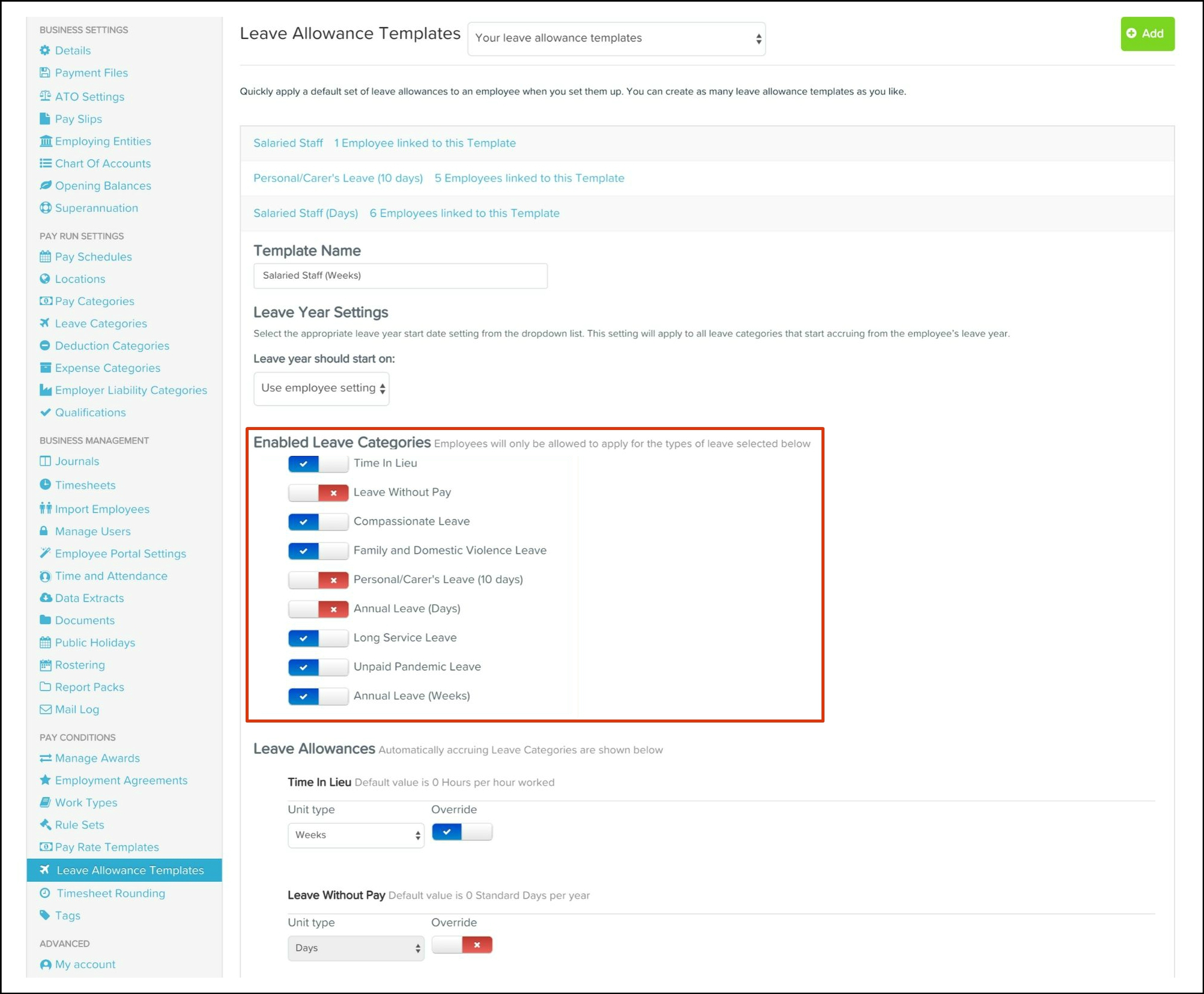The screenshot features a section titled "Leave Allowance Templates." It allows users to efficiently apply default leave allowances to employees during their setup. Users can create multiple leave allowance templates as needed. The existing templates shown include:

1. **Salaried Staff**: One employee is linked to this template.
2. **Personal/Career's Leave**: Ten days, with five employees linked to this template.
3. **Salaried Staff Days**: Six employees are linked to this template.

A new template in progress is labeled "Salaried Staff Weeks." The leave year setting requires selecting the appropriate leave year start date from a dropdown list. This setting will apply to all leave categories starting from the employee's leave year, with the default being "Use employee settings."

A highlighted red rectangle emphasizes the "Enabled Leave Categories" section, indicating that employees can only apply for selected types of leave. The options, each marked with a blue checkmark, include:

- Time in Lieu
- Compassionate Leave
- Family and Domestic Violence Leave
- Long Service Leave
- Unpaid Pandemic Leave
- Annual Leave

This detailed interface ensures that leave allowances are managed efficiently and tailored to the specific needs of both employees and employers.